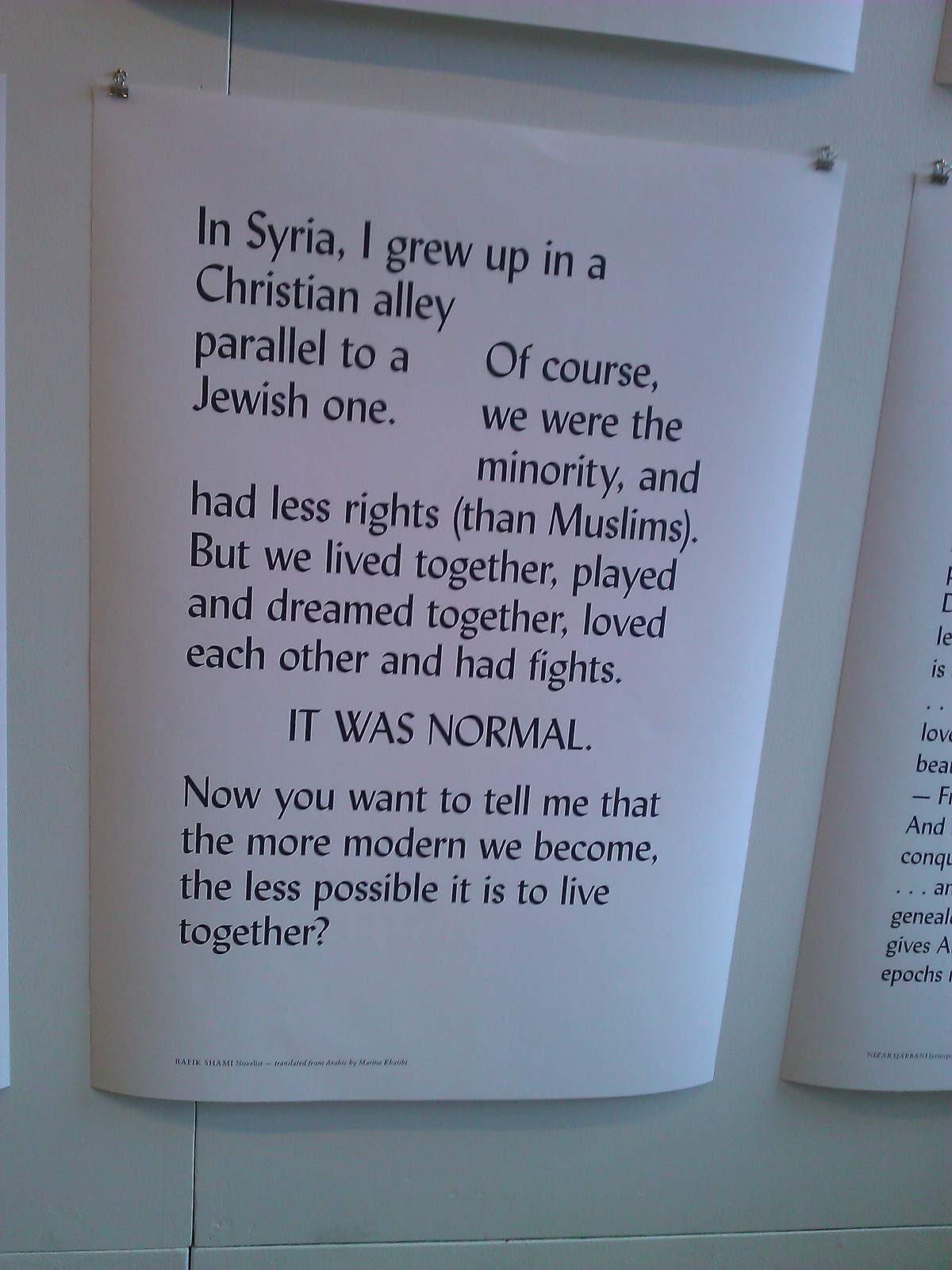The photograph displays a rectangular white piece of paper pinned to a white wall, situated among other partially visible papers, creating a grid-like display. The focal paper features a poignant text in black letters, recounting: "In Syria, I grew up in a Christian alley parallel to a Jewish one. Of course, we were the minority and had fewer rights than Muslims. But we lived together, played and dreamed together, loved each other, and had fights. It was normal. Now you want to tell me that the more modern we become, the less possible it is to live together?" Below this main text, smaller writing at the bottom credits Balik Shami, a novelist, with the translation by Marina Khalibi. This document appears to be part of a larger collection of similarly styled written anecdotes.